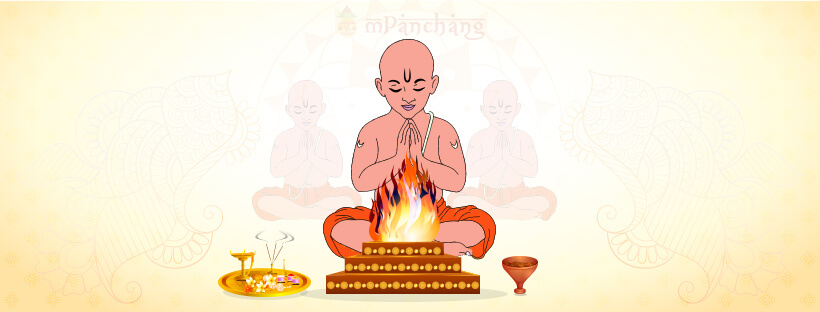This image is a detailed, animated drawing centered on a figure resembling a baby Buddha, seated in a meditative pose. The Buddha, depicted with pink skin, sits with legs crossed – the right leg wrapped over the left, and the left leg tucked under. His eyes are closed, creating a serene expression, and his hands are folded in a prayer gesture at his chest. Above his nose is a distinctive dark U-shaped mark, and draped over his left shoulder is a white strap running down his body. He wears dark orange pants that stop at his knees, leaving his upper body bare.

He sits in front of a three-tiered platform, colored in shades of brown and gold, with each tier adorned with alternating small and large yellow dots. Rising from the platform is a vivid flame with a white core, expanding outward in yellow and orange hues, reaching just below the Buddha’s folded hands.

To the left of the flaming platform lies a golden plate filled with various prayer materials, potentially including a glass and food items. On the right side is a dark brown, funnel-like object, which resembles a brass goblet with a thin stem and wider cup.

The background is a light brown hue, and faded, smaller duplicate images of the central figure appear to the left and right. At the top middle of the image, the text "M Panchang" is written faintly. Additional faint symbols and potentially images of faces or animal heads are scattered across the left and right areas of the backdrop, adding to the intricate detail of the drawing.